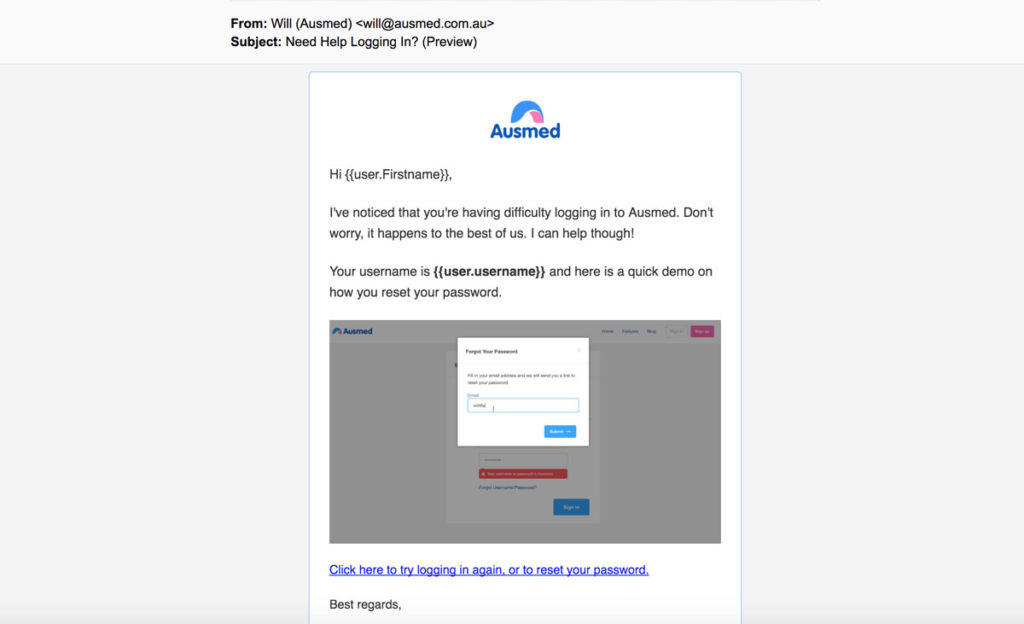The image in question is a layered screenshot featuring an email, and within that email, there exists another screenshot. The primary screenshot is an email interface with the subject line "Help, need help logging in?" displayed prominently in black and lighter grey text at the top. It originates from "will (Ausmed)" with the email address "will@ausmed.com.au."

In the central portion of the image, there's a grey box containing another screenshot showcasing a white page with the header "Ausmed" highlighted in blue. Below, the message begins with a friendly greeting, "Hi [First Name]," indicating personalization. The email continues, addressing the recipient’s issue with logging in by assuring them with a reassuring tone: "I've noticed that you've been having difficulty logging into Ausmed. Don’t worry, it happens to the best of us. I can help though!"

Following this, the user's username is displayed in a darker font: "Your username is [user.username]." The email then offers a solution to reset the password, leading into another screenshot. This embedded screenshot presents the "Forgot Password" page, where users can input their email address to request a password reset. Though the text is not fully legible, it clearly guides the user to the input field and a blue submit button.

At the bottom of the email, in blue, it provides a clickable link: "Click here to try logging in again or to reset your password." It concludes with "Best regards" in black text, marking the end of the email.